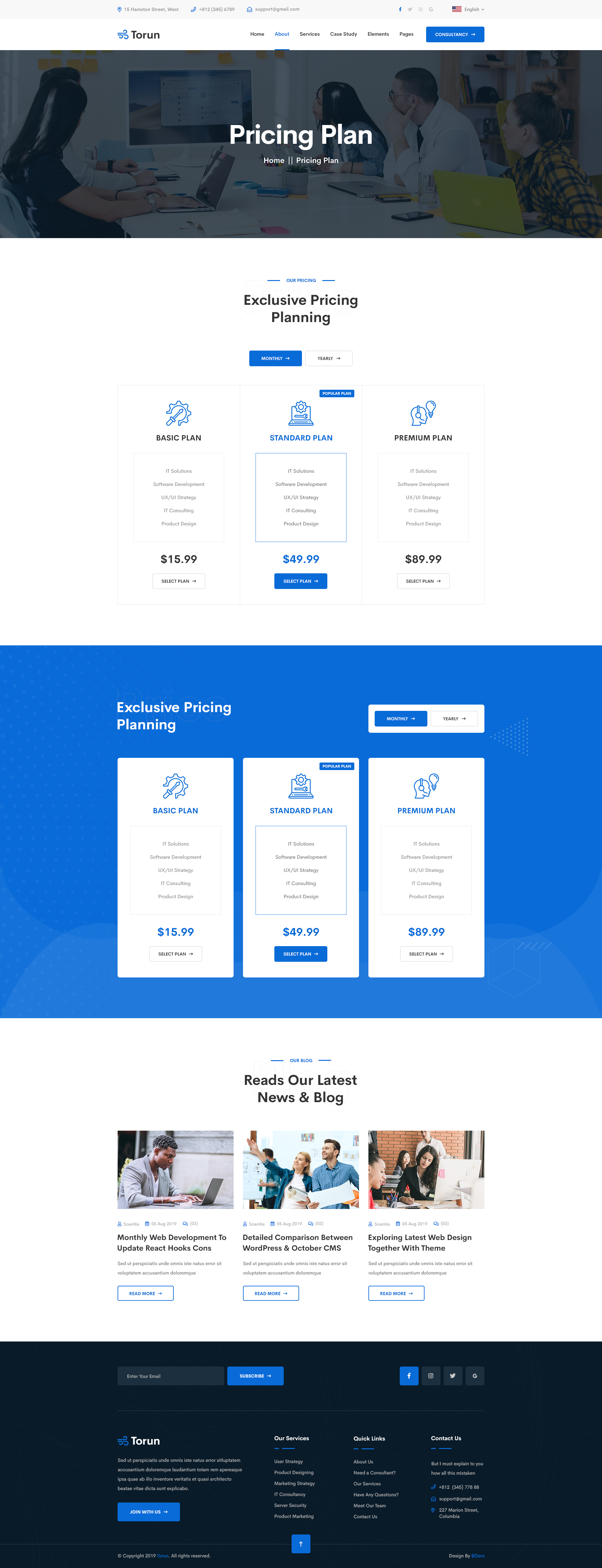The image depicts a zoomed-out view of a website interface, providing limited but discernible details. At the top, three browser tabs are visible, and on the far right corner, there appears to be a language setting option, possibly represented by the United States flag. The website name is partially visible, starting with a "T", and might be "Toru" or something similar.

Just below the website's banner, a white text bar in the center reads "Pricing Plan" over a semi-transparent black background. This section seems to overlay an image of a conference room, which includes a TV screen, a table, and at least four individuals: a lady on the left, and on the right, another lady, a man, and possibly another lady.

Further down, a white section displays the text "Exclusive Pricing Plan," accompanied by blue and white buttons beneath it. The website then showcases three pricing tiers from left to right: the "Basic Plan" at $15.99, the "Standard Plan" at $49.99, and the "Premium Plan" at $89.99. Following this, another blue section reiterates the same pricing plans with similar text.

A subsequent white section encourages visitors to "Read Our Latest News and Blog" and highlights three segments. The first segment features a man typing on a laptop outdoors, the second displays a few workers inside, possibly taking a selfie, and the third shows a woman at her computer in a setting with a red brick wall, which could be either an office space or a school.

At the very bottom, a black section presents several navigation options, resembling a search browser for the website, though the text is too small to discern clearly.